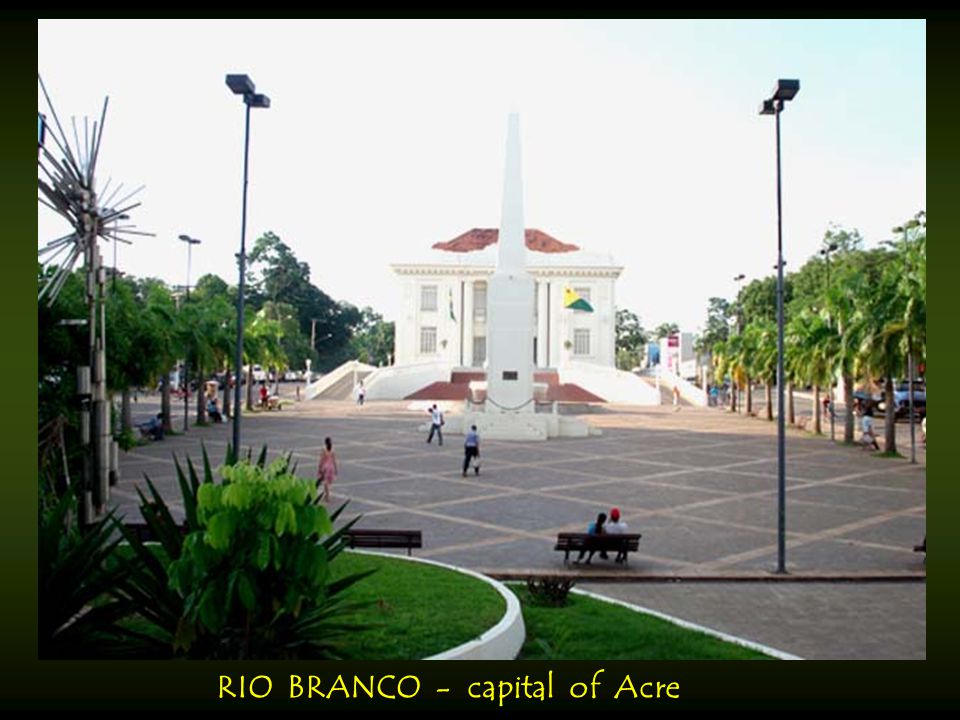The image resembles a postcard with a dark green outer border and gold lettering at the bottom center, labeled "Rio Branco - Capital of Acre." At the heart of the image stands a tall, white statue that narrows towards the top, set in the middle of a paved courtyard. This courtyard, separated into gray and brown squares outlined in a lighter color, is surrounded by green palm trees and park benches. People can be seen walking and sitting in the area. Behind the statue is a white building with a terracotta roof and white stairs on either side, likely a museum. Two streetlights frame the scene symmetrically, providing a sense of balance to the daytime view captured in this tranquil square.